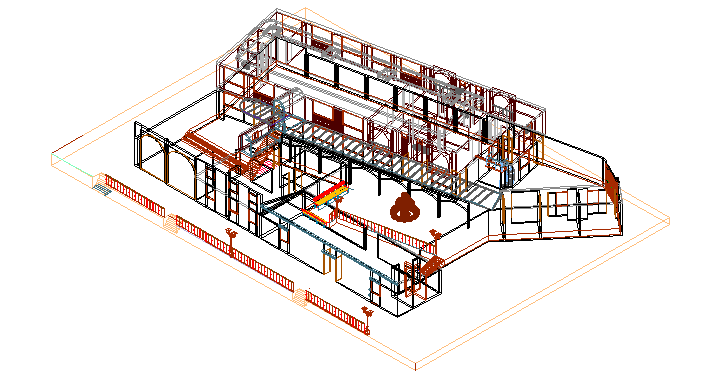The image depicts a wireframe computer rendering of a large, possibly industrial building, with no background. Dominated by a palette of silver, brown, maroon, orange, red, and yellow, the 3D model showcases a cluttered and intricate design, characterized by numerous intersecting lines in predominantly orange and black hues. The structure itself is diagonally shaped and rectangular, with multiple visible sectors and at least two to three stories. Notable features include several ladders, indicative of multiple levels, and a prominent red fence on the left-hand side, extending from the top left diagonally to the bottom right. The fence alternates in shades of red and dark red, interspersed with elements that might represent stairs or additional fencing. The building appears transparent, with visible outlines of windows and a possible entrance, contributing to the complex and somewhat confusing visualization.